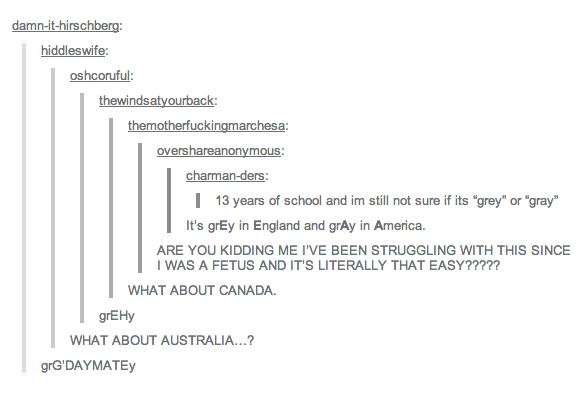The image depicts a set of comments on a forum or social media post, presented in a unique and somewhat confusing layout resembling a sideways pyramid. The initial comment at the "top" of this pyramid starts a discussion about the correct spelling of the color grey/gray, with the original poster expressing frustration over not knowing whether it's "GREY" or "G-R-A-Y" after 13 years of schooling. 

Following this, the conversation branches out with users providing input, clarifying that "GREY" is the preferred spelling in England, while "GRAY" is commonly used in America. The ensuing comments include various expressions of long-standing confusion over the issue, with one user humorously lamenting their struggle since birth. As the discussion continues, others inquire about the spelling conventions in Canada and Australia.

The usernames of the commenters add a layer of eclectic humor and personality, featuring names such as "Hitler's wife," "the motherfucking March ESA," and "the winds at your back." These names appear on either side of the comments they correspond to, adding further to the complex visual structure of the image.